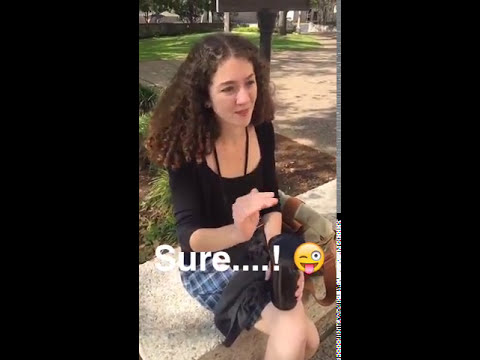The image depicts a young white woman with very curly, shoulder-length hair, sitting outdoors on a stone or concrete bench. She is dressed in a black three-quarter-sleeved top with a deep, round neckline that exposes her shoulders and part of her chest, complemented by a blue plaid short skirt. She wears red lipstick and is seen holding a dark-colored cup in one hand while a dark jacket or sweater rests across her lap. Around her neck, partially obscured by her hand, is a cord, the purpose of which is unclear. To her right (left in the image) sits a tan purse with brown straps. The scene is bathed in daylight and text on the bottom of the image reads, "sure....!" followed by a winking tongue-out emoji.